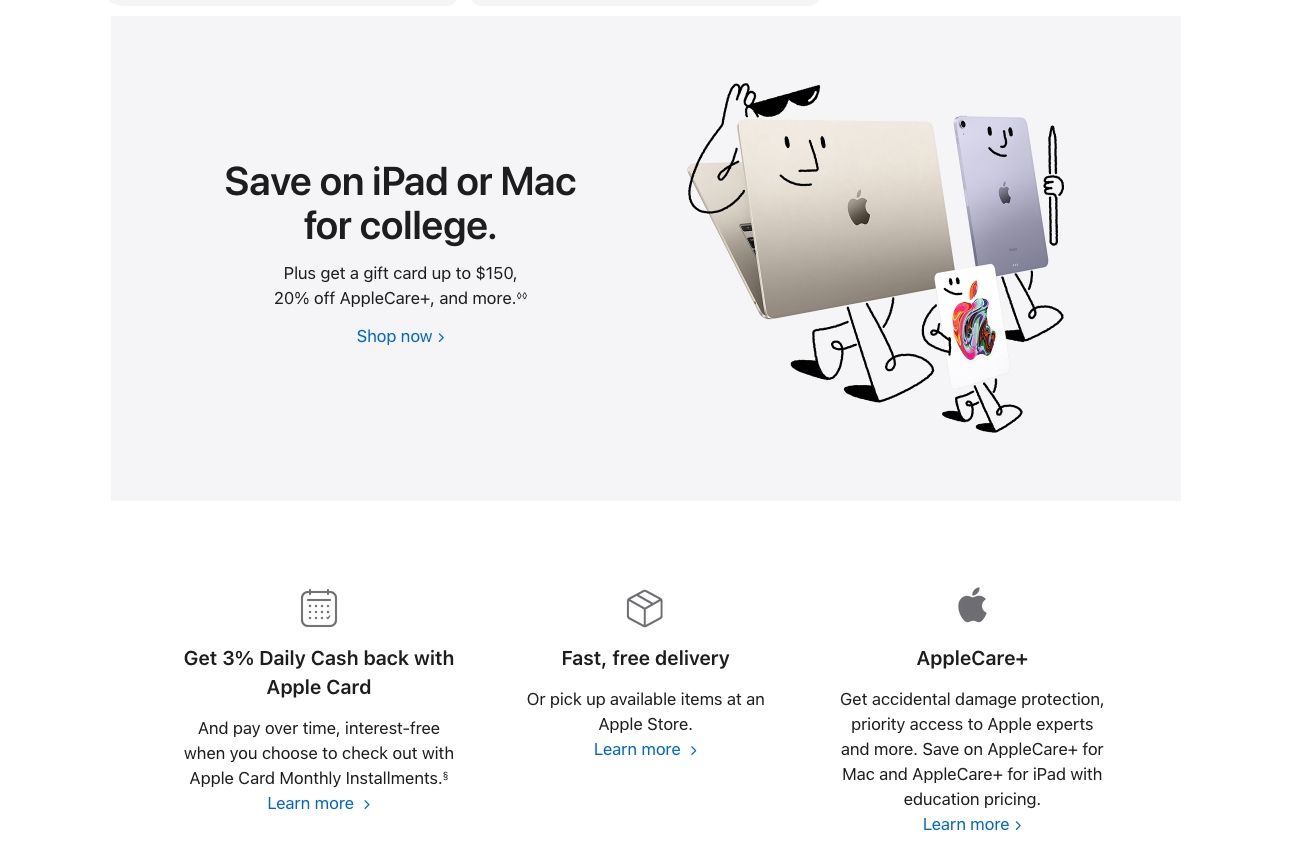**Screenshot Description:**

At the top of the webpage, there is a whimsical illustration featuring a laptop, an iPad, and a gift card, each adorned with playful, cartoon-like faces. The laptop sports sunglasses, held by a drawn arm extending to the right, and both the laptop and iPad have small feet illustrated beneath them. Additionally, there is a gift card (initially mistaken for a phone) with a face encircled by an Apple logo in the center, though its white coloration blends into the whitish background. 

Above the gadgets, a text banner reads: "Save on iPad or Mac for college. Plus, get a gift card up to $150. 20% off Apple Care+ and more." 

Below this banner, the website is organized into three distinct columns:
1. **Get 3% Daily Cash Back**: Describes the benefit of receiving 3% daily cash back with the Apple Card and mentions the option to pay overtime, interest-free, via Apple Card monthly installments.
2. **Fast, Free Delivery**: Promises a quick and cost-free delivery service.
3. **Apple Care+**: Highlights the availability of Apple Care+ for additional protection and support.

The detailed design and information convey a sense of fun while presenting the promotional offers and benefits clearly.